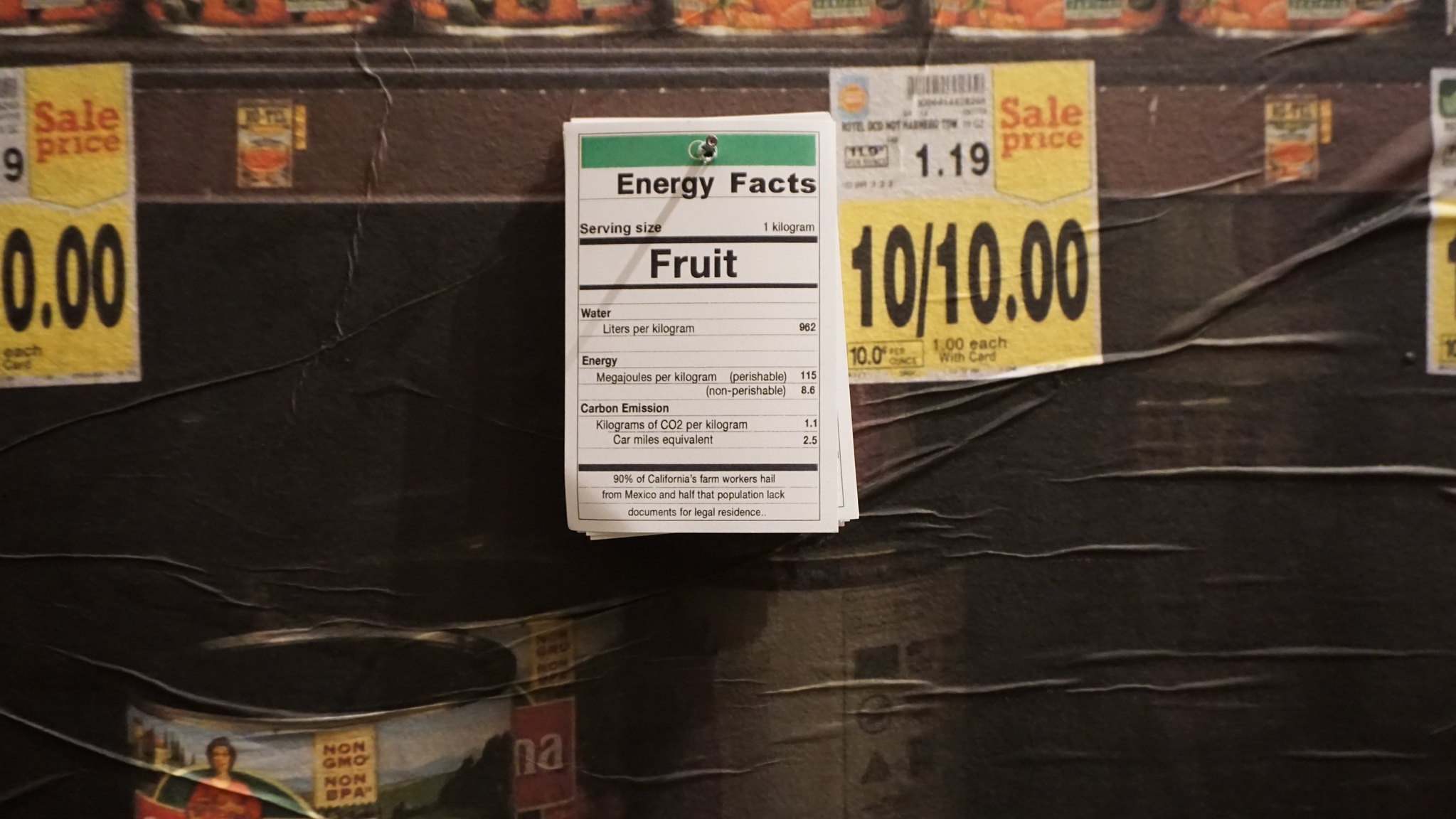This image, at first glance, appears to depict shelving inside a grocery store, showcasing familiar elements like price labels, plastic shelving edges, and rows of tin cans of Rotel fruits and vegetables, some partially out of frame. Upon closer inspection, however, it becomes clear that this is not an actual photograph taken inside a store. The image is instead a high-quality print, likely a poster or wallpaper, that mimics the scene of a grocery aisle. This illusion is disrupted by noticeable imperfections: wrinkles and a tear run across the shelves and products, particularly visible on the right side of the image where long bubbles and ripples distort the flat representation. Additional details include a brown-themed background with signs of wear, such as paint chipping, and a texture suggestive of damage. The imagery includes sale prices with regular prices listed as $1.19 and a sales promotion of 10 cans for $10, highlighted in red font with a downward arrow. Small cards pinned with pushpins provide energy facts for the fruits, displaying information on serving size, water, energy, and carbon emissions. The scene, though convincing at a casual glance, reveals its true nature through these textual irregularities and physical distortions.